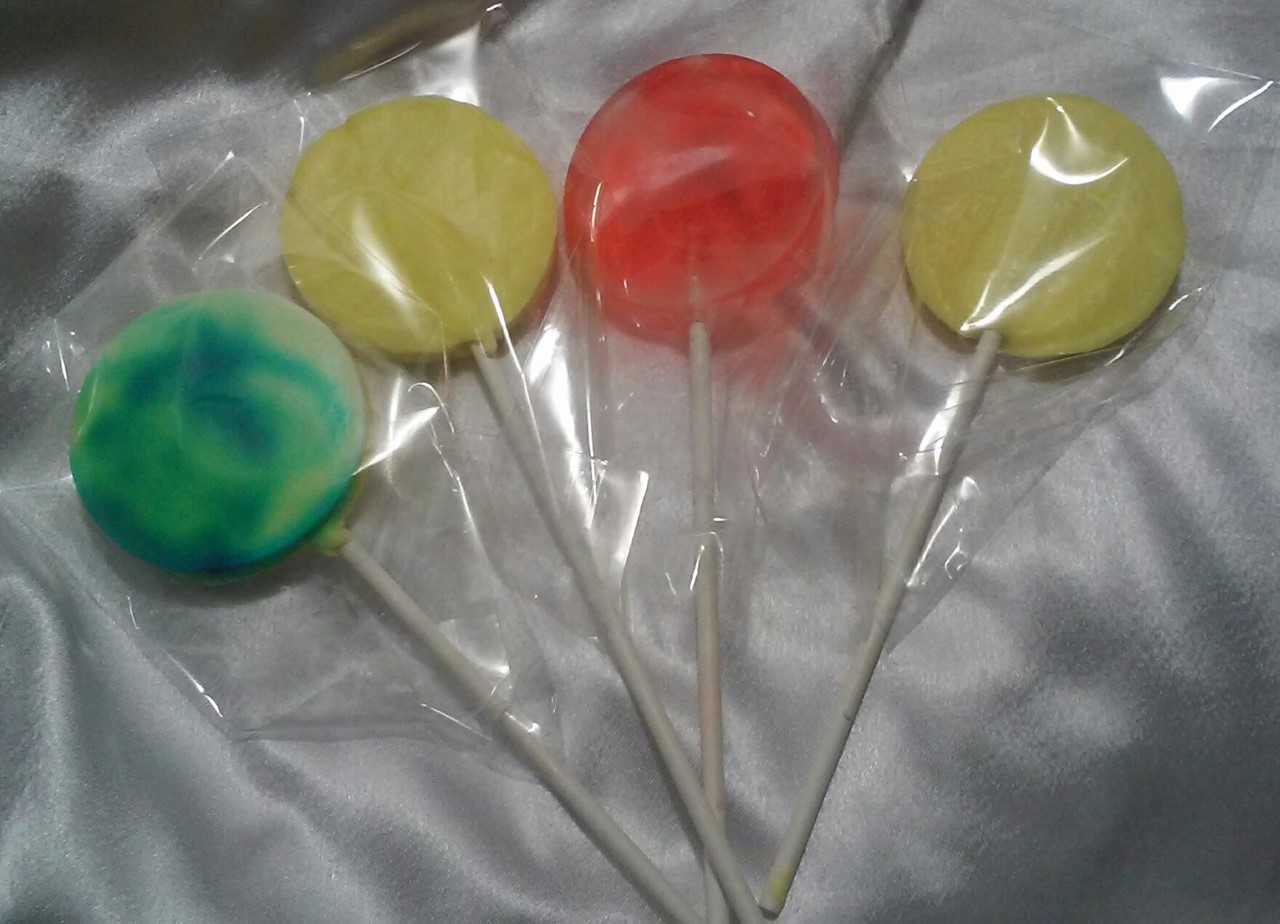The digital photograph, taken indoors, features a piece of wrinkled, off-white or gray fabric as the backdrop. At the center of the image, four round lollipops are arranged in a flared pattern, with their white sticks facing towards the camera and fanning outwards. Each lollipop is individually wrapped in thin, clear plastic, which catches some light reflection. From left to right, the lollipops are as follows: the first has a green and turquoise swirl pattern, the second is solid yellow, the third is solid red, and the fourth is another solid yellow. The entire photo is in a square format, emphasizing the textured fabric and colorful lollipops.